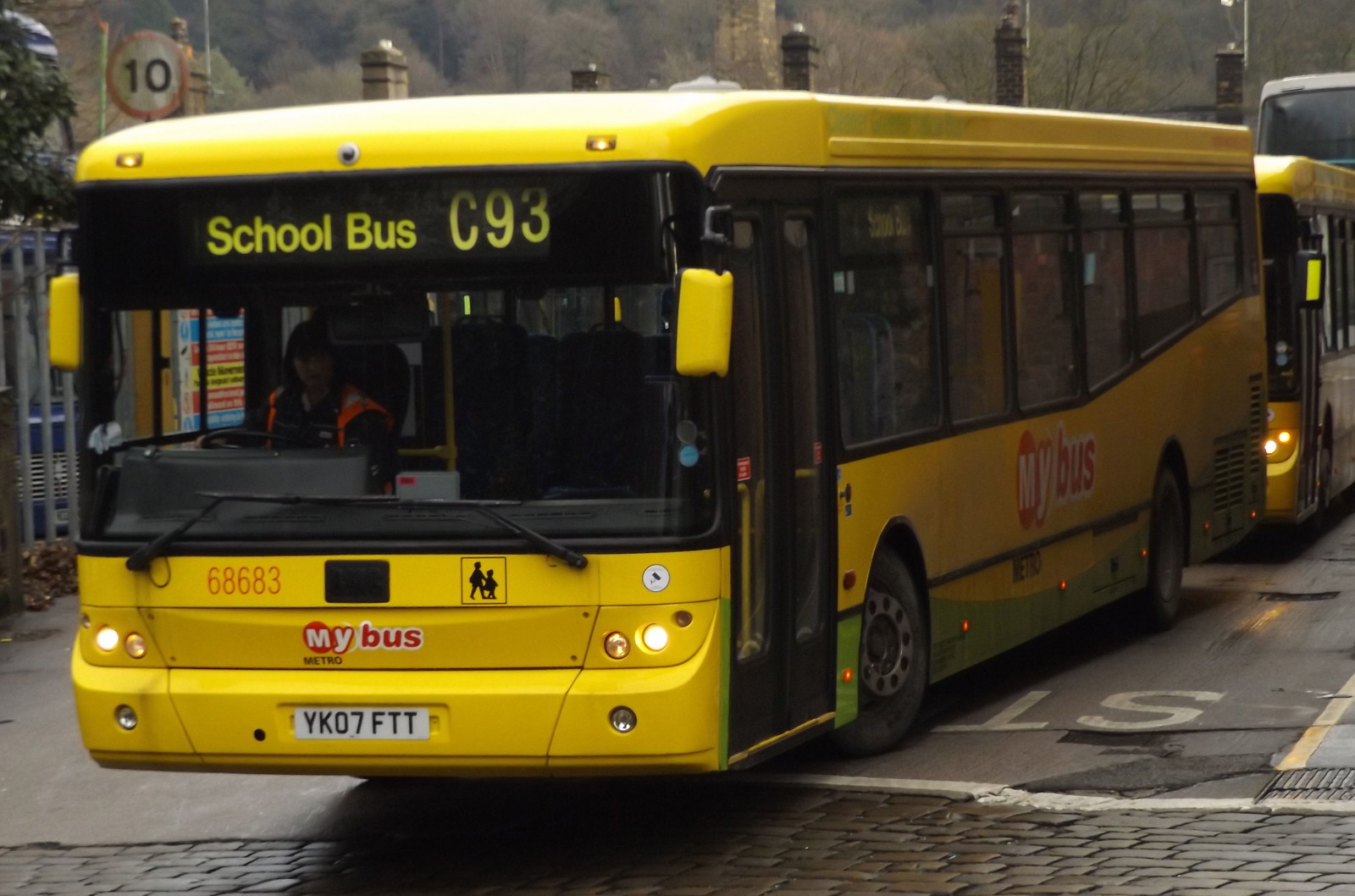The photograph captures a vivid scene of two modern, bright yellow school buses on a cobblestone street. The foremost bus, prominently displayed, features a white European license plate with the text "YK07FTT." At the front, in large yellow adjustable letters on the windscreen, it is identified as "SCOBUS C93." Just below the windshield, bold red numbers "68683" further identify the vehicle. A distinct "my bus" logo in white writing, surrounded by a red circle around the "M" and "Y," is also visible, adding a touch of personalization to the bus. Seated on the right-hand side of the front bus, the driver is noticeable in an orange and yellow safety vest paired with a black jacket. The headlights of the bus are modern, with small, likely LED or halogen lights, indicating the bus's contemporary design. In the background, there's a second yellow school bus closely following, and further beyond, trees and chimneys are visible, cementing the scene in a quaint yet urban environment.